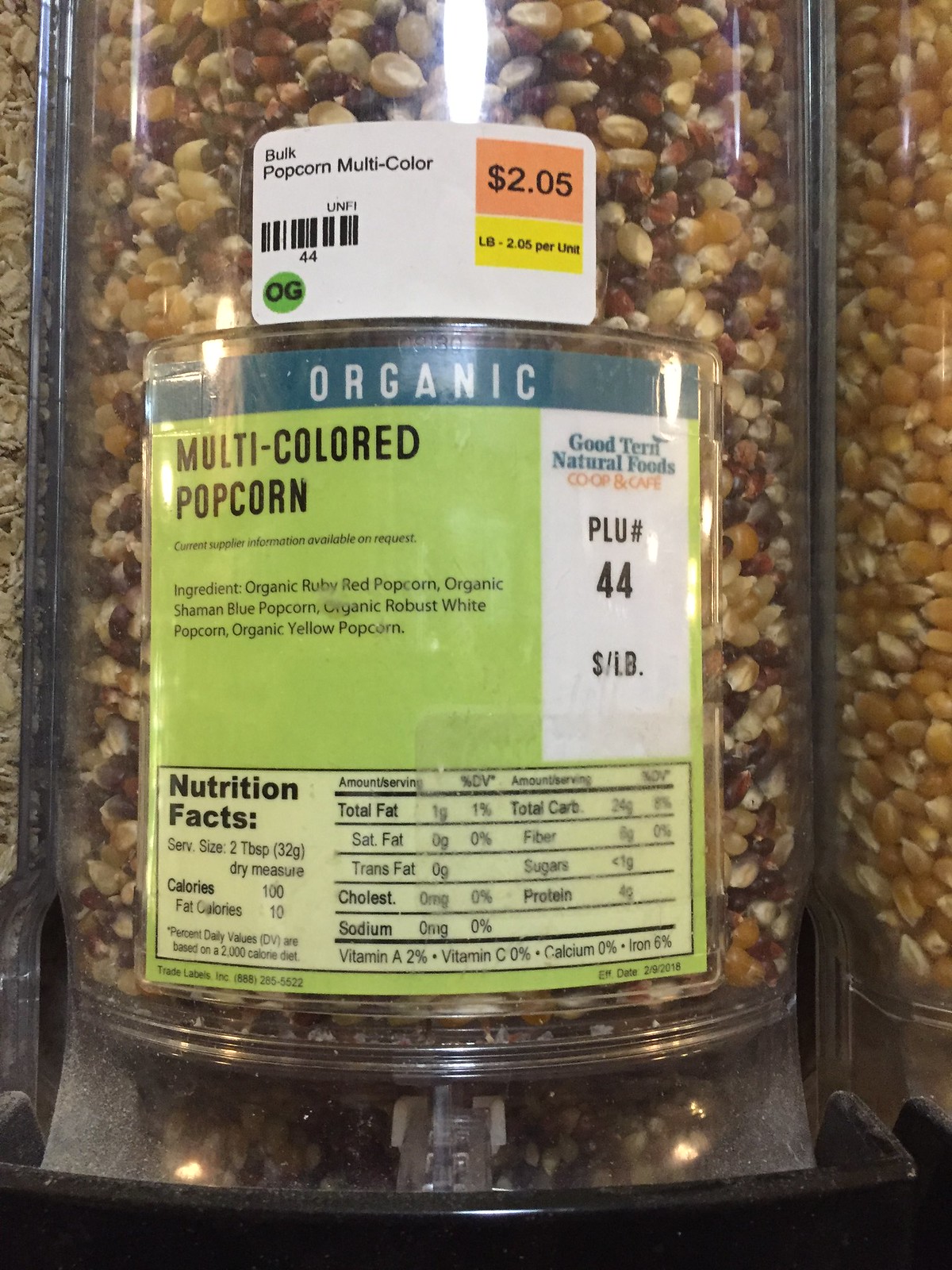A detailed caption for the image:

In the image, there is a clear plastic container of multicolored popcorn kernels prominently displayed, part of a bulk section in a grocery store. This container, designed for customers to fill their own bags, is flanked by another container of plain popcorn kernels on the left and a container of sunflower seeds on the right. The popcorn kernels inside the main container are a vibrant mix of reds, blues, whites, and yellows, filling the bin almost to the top. 

At the top center of the container is a white label with black text that reads "Bulk Popcorn Multicolor." Below this, in an orange box, is the price "$2.05," and directly underneath, in yellow, it specifies "per pound, $2.05 per unit." A barcode is also present with the notation "UNFI" or perhaps "UNF1" followed by the number "44." A green circle with the letters "OG" is prominently displayed, indicating the organic nature of the product.

Beneath the white label is a dark green label with white text. The top portion states "Organic." The text below reads "Multicolored Popcorn," followed by "Current supplier information available on request" and a list of ingredients: "Organic Ruby Red Popcorn, Organic Shaman Blue Popcorn, Organic Robust White Popcorn, Organic Yellow Popcorn." Along the side of this label, it mentions "Good Term Natural Foods, CD-CP and Cafe, PLU number 44, price per pound." Additionally, there are nutrition facts displayed at the bottom of the label. The design transitions into a lighter green section at the very bottom.